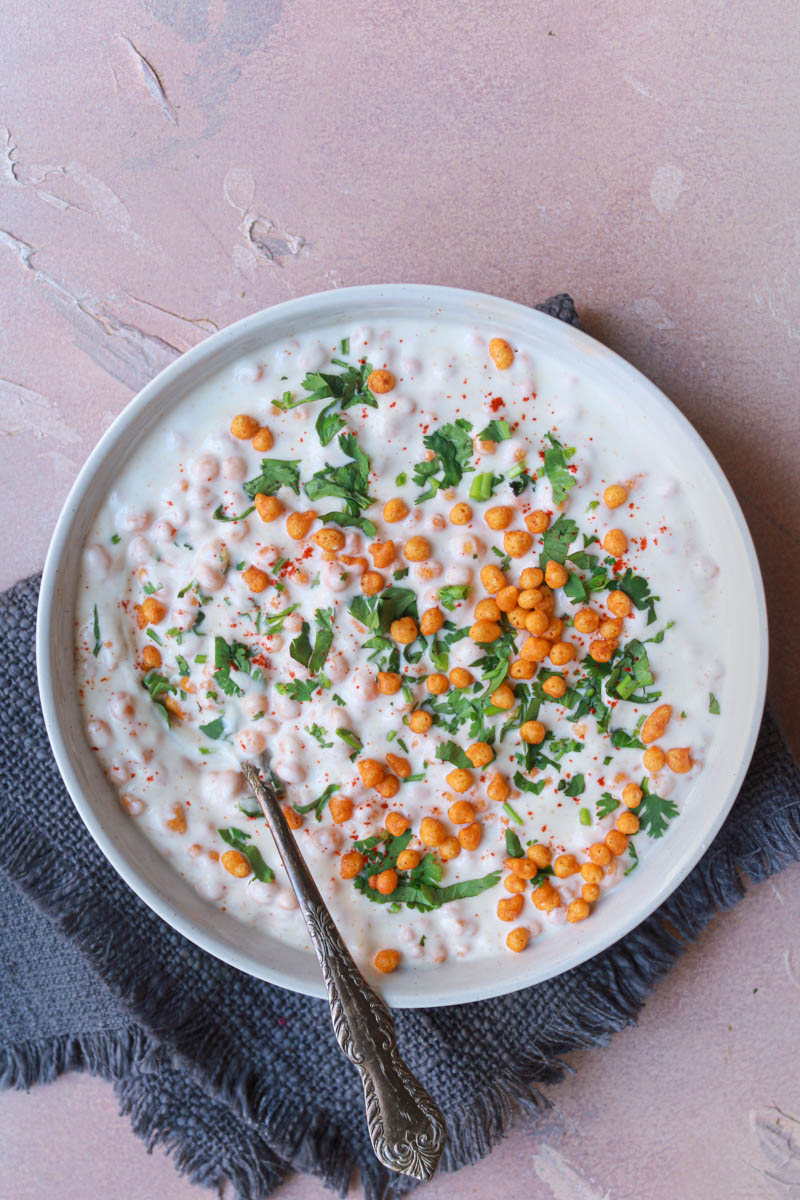A meticulously arranged culinary scene captures a white ceramic bowl filled with a thick white creamy mixture, possibly yogurt or soup, adorned with small orange pellets, likely chickpeas, and green garnish, such as basil leaves or parsley. The bowl sits atop a deep blue-gray fringed napkin with visible woven strands, while a silver spoon rests on its left side. This setup is placed on a table featuring a textured pink surface, embellished with splotchy lavender, blue, and white streaks. The overall image is balanced and visually appealing, showcasing both the intricate details of the dish and the artistic backdrop.